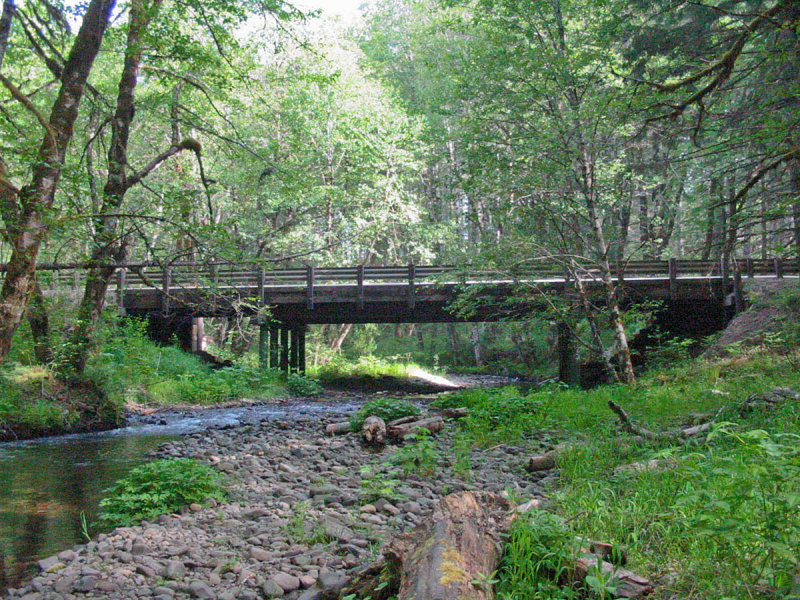This color landscape photograph captures a professionally built, uniformly constructed wooden bridge spanning a shallow stream in a lush woodland area during daytime in either spring or summer. The bridge, positioned about 50 yards ahead, appears dark brown and gray, supported by two sets of pillars. It features railings on either side. The stream, emerging from the left side of the image, meanders towards the center and flows under the bridge, which stands clearly in the background amidst a densely packed forest with trees boasting light green leaves. The foreground includes gray and beige rocks, a fallen tree trunk, and a variety of plants, depicting a richly vegetated scene with grass and greenery on the ground, enhancing the realism and natural beauty of the setting. Some fallen logs and trees partially obscure the view of the bridge, giving the photo a sense of depth and immersion in the natural environment.